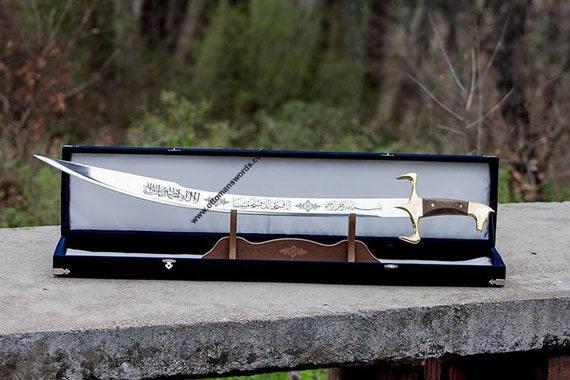The image depicts a long, curved ceremonial or art knife, prominently displayed outdoors during the daytime against a natural backdrop of trees and bushes. The knife is elegantly set on a gray concrete slab or bench, lying within an open dark blue case lined with white velvet, and placed on a slightly elevated wooden pedestal. The hilt of this intricate piece features a combination of gold and brown, possibly made of wood, enhancing its ornate design. The shiny silver blade is adorned with detailed engravings that appear to be in Arabic, alongside a small artistic design. A small, inconspicuous copyright watermark is also visible, and the blade bears the website address "www.ottmansworlds.com."